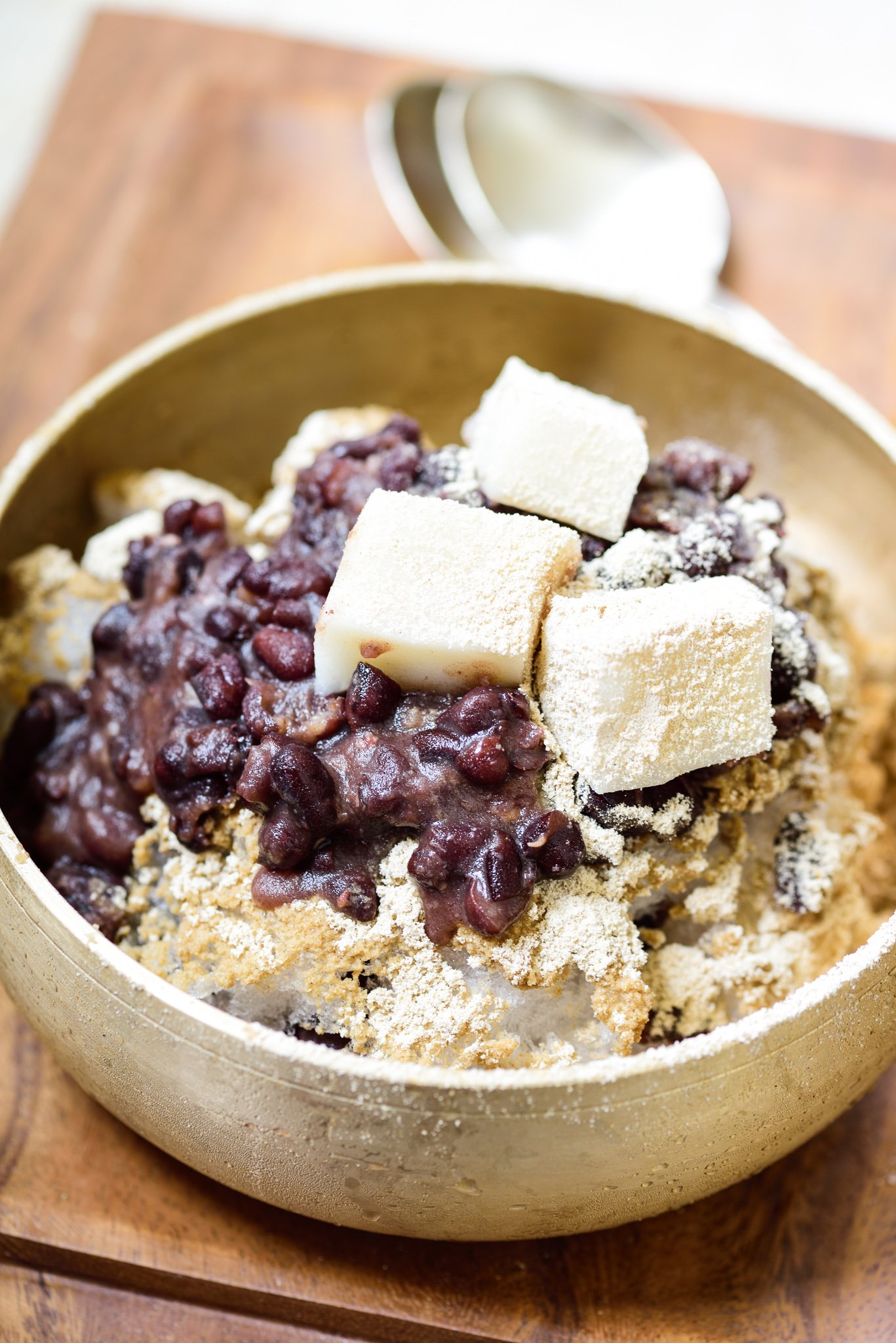The image features a close-up, portrait-mode view of a rustic dining setup. At the center is a tan, wooden bowl, approximately two-thirds the size of a standard cereal bowl, placed on a medium brown, wood-textured square tile. In the background, two blurred tablespoons can be seen, overlapping slightly in the upper-right corner. The lighting comes from the lower right, illuminating the contents of the bowl. Inside the bowl is a crumbly, brown-base dish topped with three cubes of butter at the center. The dish also features dark purple, oval-shaped items, possibly beans or blueberries, in a purplish sauce on the left side. The overall appearance suggests a breakfast item, potentially a biscuit with a blueberry jam topping. The bowl contrasts with the darker brown tray, enhancing the rustic, cozy ambiance.